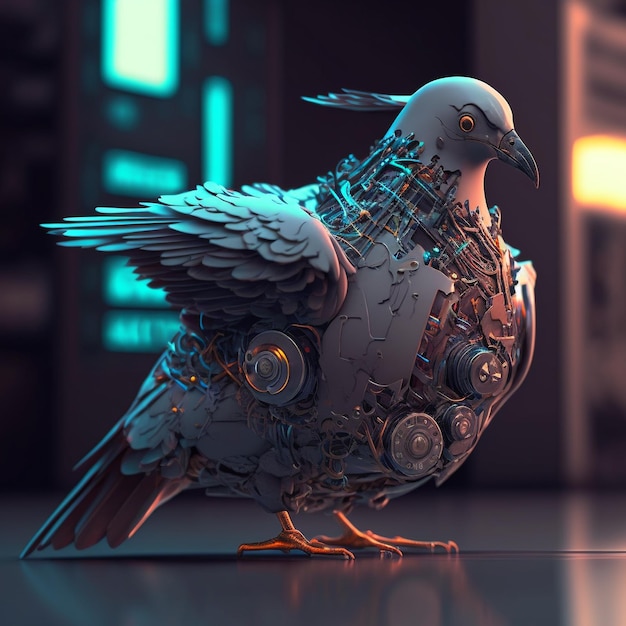The image features a highly detailed digital artwork of a robotic pigeon, centrally positioned and facing slightly right. This robotic pigeon is portrayed with a gray metallic body, and its head is distinctly pigeon-like with a black beak and striking golden eyes. The pigeon’s body showcases exposed mechanical components, including gears, disks, and an intricate network of wires, which can be seen particularly around and beneath the neck.

Notably, the chest area reveals circular metallic pieces, while the right side of the body, below the wing, contains another circular component with visible wires threading through it. The wings and tail feathers are also meticulously rendered, appearing to be made of a grayish-blue metal. The wings extend outwards, and beneath them are more intricate details, such as gold and blue wires.

The bird stands on a gray, reflective surface with its dark orange legs and feet firmly positioned. The background is artistically blurred, highlighting two main sources of light: an orange-yellow light on the right and a blue light on the left, along with some indistinct gray structures. This composition captures the blend of mechanical intricacy and avian form, embodying a futuristic, metallic essence against a soft, diffused backdrop.